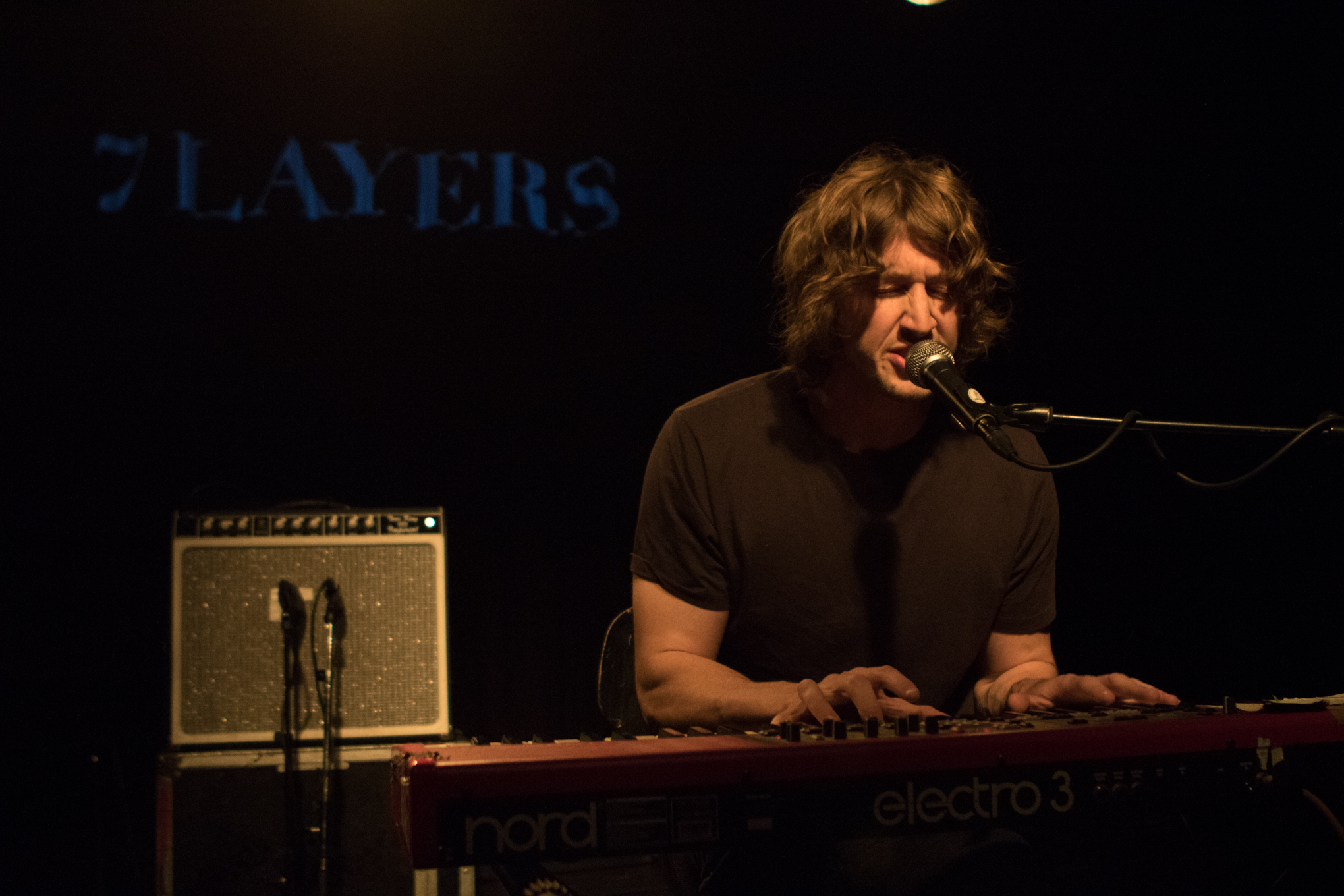The photograph features a man with long, dark hair that curls slightly at the ends, seated at a red Nord Electro 3 keyboard. His hands are spread out over the keys as he performs, eyes closed, singing into a black wired microphone that extends from the right side of the frame. The man, who is centered in the image, is illuminated by a soft amber light, highlighting his black short-sleeved shirt. In the background, which is predominantly dark, there is faint blue lettering above him that reads "seven layers." To his right, a piece of equipment featuring wires can also be seen. The black buttons on the keyboard add intricate details to this captivating musical scene.